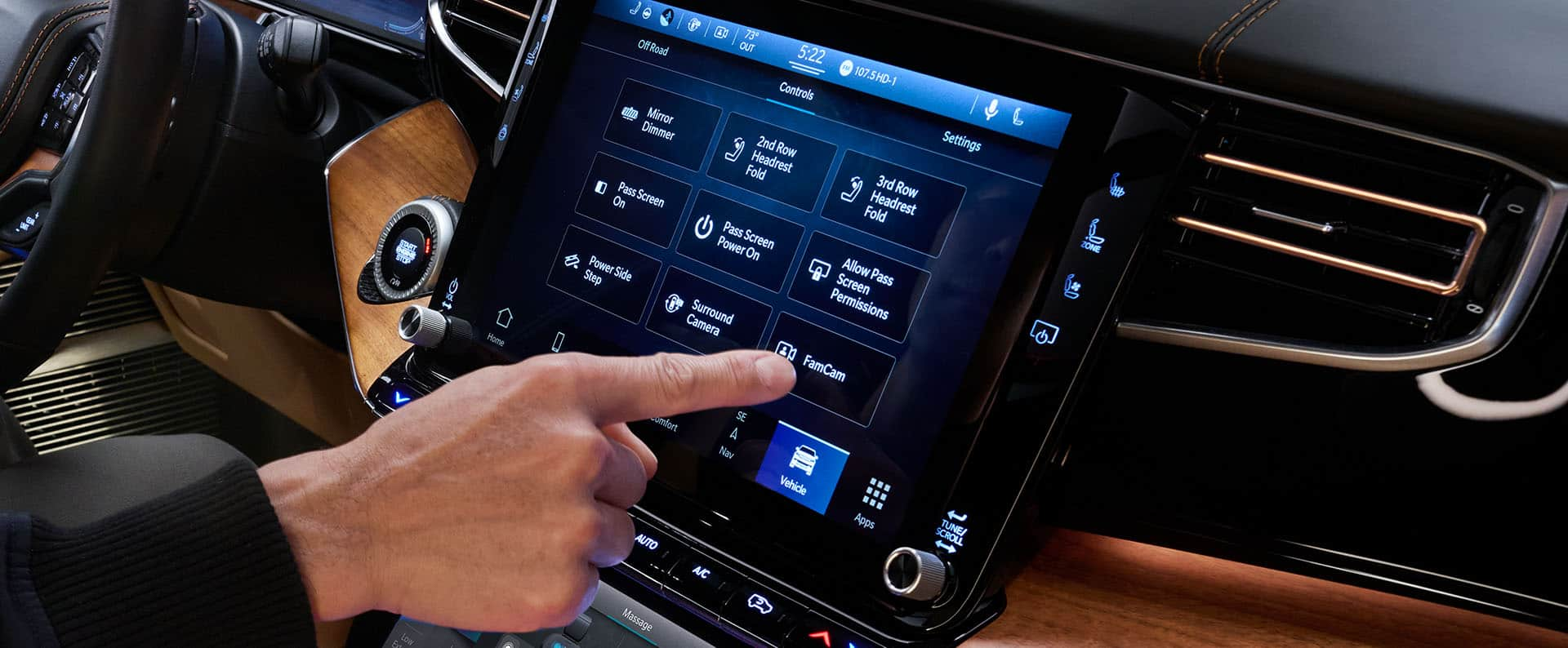The photograph captures an interior view of a car, focusing on the central GPS or communication center screen. A Caucasian individual, wearing a black shirt, is depicted touching one of the screen's options labeled "Face Cam." The screen is bordered by a blue bar at the top and displays several rectangular choices. In the upper left corner, part of the steering wheel is visible. The dashboard features a wood grain finish with a silver button or knob towards the left, complemented by black leather with silver trim on the upper section. On the computer screen, additional settings such as seat controls and a power button are observable, along with another silver knob in the corner. The entire setup underscores a seamless blend of technology and luxury within the vehicle's interior design.